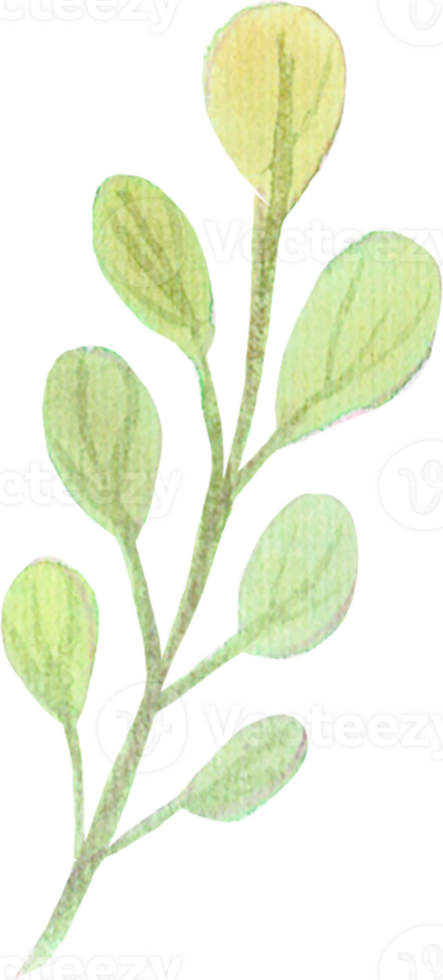The image depicts a simple, vertically oriented pencil drawing of a single green plant with a thin, slightly darker grayish-brown stalk. This main stem has branching stems on either side, each bearing three uniformly shaped, teardrop-like leaves, adding up to six lateral leaves in total. At the apex of the stalk, there's an additional solitary leaf, slightly more yellow than the others. Each leaf features clearly illustrated veins, approximately three per leaf, contributing to a detailed yet basic botanical depiction. The overall coloration of the leaves is a very light, pale, mint or sage green, suggestive of colored pencil work. The entire visual carries a rudimentary charm with its light pigment and straightforward structure.